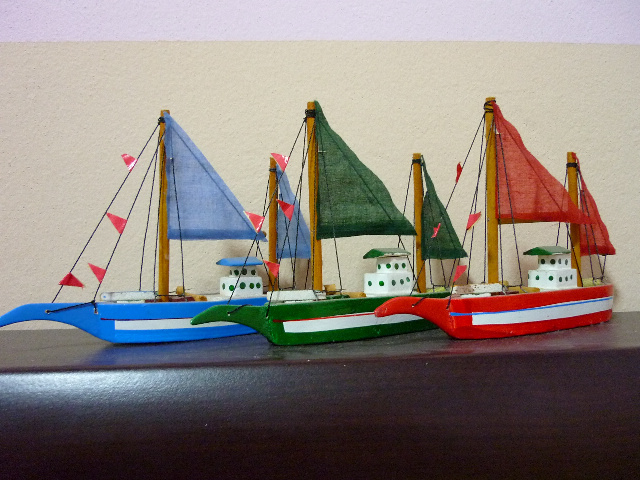This photograph captures three neatly arranged model boats, each with distinct colors and simple, old sailboat designs, positioned from left to right on a mahogany-colored table. The first boat features a blue hull and sail, with red flags adorning the rigging and a matching blue roof on its white wheelhouse. The middle boat displays a dark green hull and sail with similar red flags on the rigging, and likewise has a green roof over its white wheelhouse. The third boat, red in both hull and sail, is accented with red flags and a green roof on its white wheelhouse. All three models are oriented sideways to the left, displayed against a cream-colored wall, creating a cohesive and visually appealing scene.